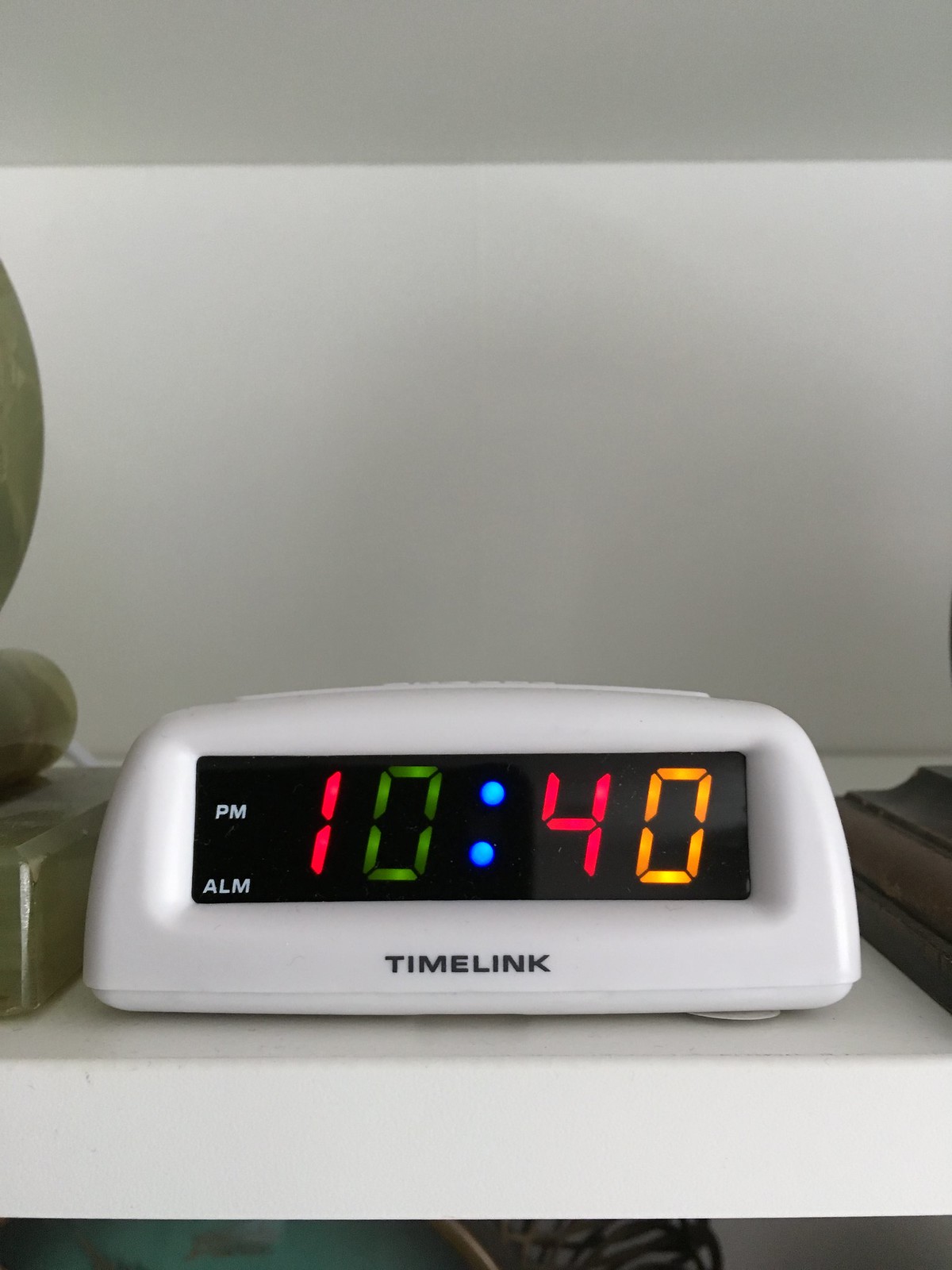The photograph shows an indoor scene with a small, white plastic digital alarm clock sitting on a one-inch thick white shelf. The clock has a rounded rectangular, almost pillow-shaped design. On its rectangular black display, multi-colored LED digits are showing the time as 10:40 PM. The digits are distinctively colored: the "1" is red, the first "0" is green, the colon is blue, the "4" is red, and the final "0" is a yellow-orange with tints of yellow. The word "TimeLink" is prominently displayed in black capital letters on the lower portion of the clock's front frame. From our low vantage point, we can just see the slight ridge of buttons on top of the clock but not how far back the clock extends. The shelf appears to have a few other ornaments on either side of the clock, and the setup is against a white wall.